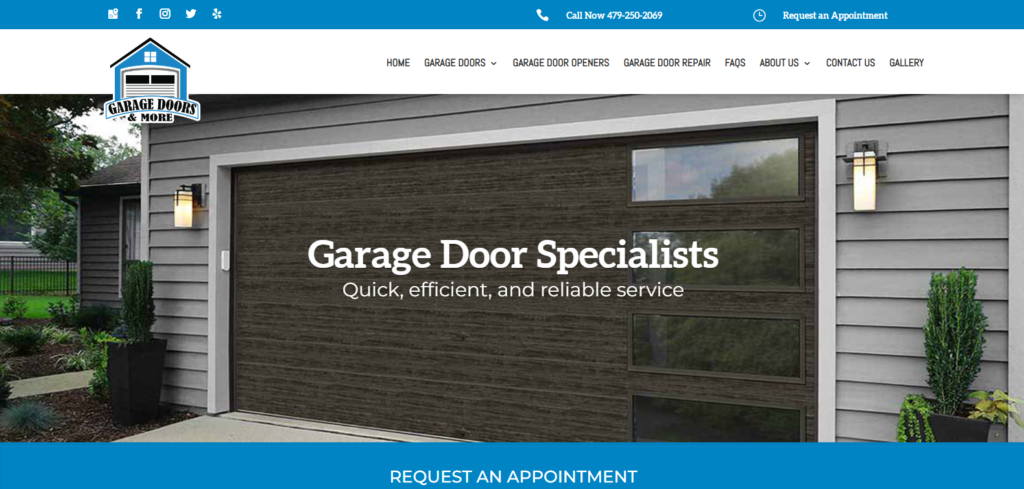The image captures a webpage from a website specializing in garage door services. At the very top, there is a hand-drawn or digitally created illustration of a blue house with the text "Garage Doors and More" prominently displayed. This section also features clickable icons for various social media platforms. A white button labeled "Call Now" is accompanied by a phone number, and there is an icon of a clock for requesting appointments.

Below this blue header area, the webpage transitions to a white section with a navigation menu located towards the center. The menu includes links to "Home," "Garage Doors," "Garage Door Openers," "Garage Door Repair," "FAQs," "About Us," "Contact," and "Gallery."

Dominating the next section of the webpage is a large, visually striking image of a home. The focal point of this image is a beautiful brown garage door with four rectangular windows aligned vertically on the right side. The text overlay reads, "Garage Door Specialist: Quick, Efficient, and Reliable Services."

Finally, at the bottom of the webpage, there is a prominent blue rectangle spanning the width of the page with a call-to-action button that says "Request an Appointment."

Overall, the webpage is designed to provide easy navigation and clear calls to action, enhancing the user experience for anyone seeking garage door services.